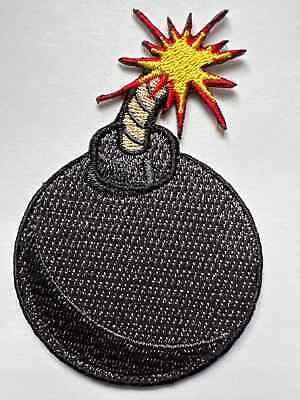The image depicts an embroidered patch designed to resemble an old-style cartoon bomb. The black bomb, spherical and reminiscent of a bowling ball, is crafted from fabric and appears textured like a shirt. Emerging from the short cylindrical top of the bomb is a thick, striped fuse, angled upwards and to the right. The fuse is beige with black stripes and culminates in an explosion effect, depicted as a yellow star with ten spikes, each outlined in vibrant red to indicate a lit fuse about to set off the bomb. The patch sits against a white background, likely a piece of paper or tabletop, and the photo itself is of a low resolution and pixelated.